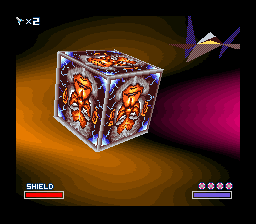This screenshot captures a low-resolution image from a video game, possibly from the Star Fox series. Dominating the center is a detailed, three-dimensional cube showing only its left, right, and top sides. The sides of the cube are adorned with an intricate orange and gray design, possibly depicting a creature or face with electrical blue sparks emanating from its corners. The top of the cube has additional gray features. In the background, an amber and magenta gradient creates a vibrant, dynamic setting.

In the upper left corner of the image, there's a symbol followed by "X2," indicating two lives remaining. A low-resolution, polygonal spaceship in blue, white, and yellow with purple wings is visible in the upper right corner, reminiscent of ships from Star Fox 64. The bottom left corner displays a fully red shield bar signifying health, with "Shield" written above it. In the bottom right corner, a purple bar with three white and red circles, and a blue bar beneath it, add further detail to the game's HUD.